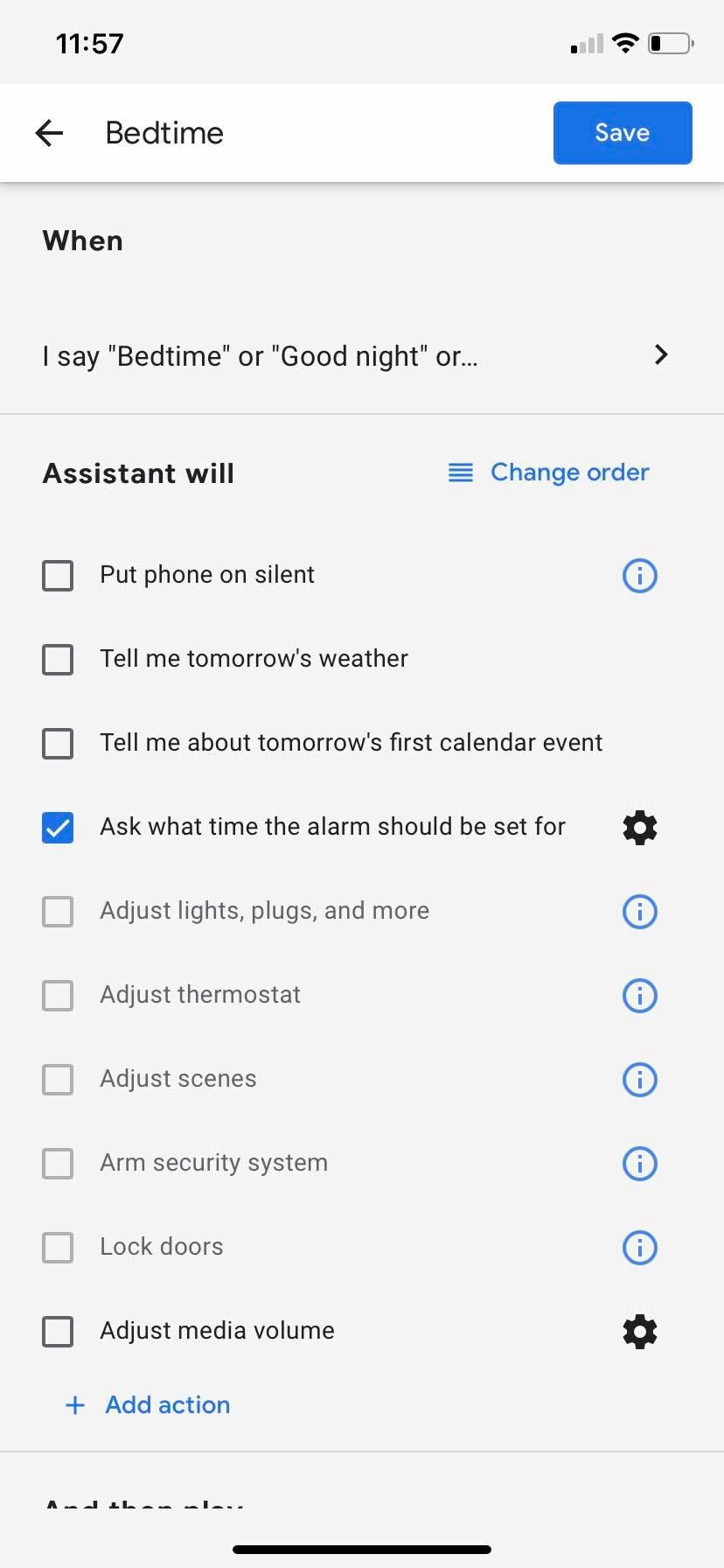Screenshot Description from a Smartphone:

This image appears to be a screenshot from an iPhone, displaying a feature likely related to bedtime settings or routines. At the very top, there's a light gray status bar with dark gray or black text indicating the time as 11:57. The status bar also shows a signal strength icon with one out of four bars filled, a fully filled Wi-Fi icon, and a battery icon that indicates less than one-third charge remaining.

Below the status bar is a white banner containing a gray back arrow on the left, gray text in the center that reads "Bedtime," and a blue button on the right with white text saying "Save."

Immediately following the banner, there is a section with a light gray background and predominantly black text. The section is labeled "When," followed by instructional text stating: "I say 'Bedtime' or 'Good night' or..." A right-facing arrow appears next to this text, followed by a separator line.

Underneath the separator, the next segment is titled "The assistant will," with blue text on the right side that reads "Change order," indicating that actions can be reordered. This segment includes a series of checkboxes with different bedtime actions and settings:

1. Unselected checkbox with the text "Put phone on silent" and an information icon.
2. Unselected checkbox labeled "Tell me tomorrow’s weather."
3. Unselected checkbox labeled "Tell me about tomorrow’s first calendar event."
4. Selected checkbox reading "Ask what time the alarm should be set for" and a settings gear icon next to it.

There are several grayed-out options that appear to be non-selectable at the moment:

1. "Adjust lights, plugs, and more."
2. "Adjust thermostat."
3. "Adjust scenes."
4. "Arm security system."
5. "Lock doors."

Near the bottom, there's a selectable checkbox (currently unselected) labeled "Adjust media volume," accompanied by another settings gear icon.

The interface concludes with a blue plus sign and text that says "Add action," followed by another separator line. The bottom of the screenshot is cut off, indicating there might be additional options or information below.